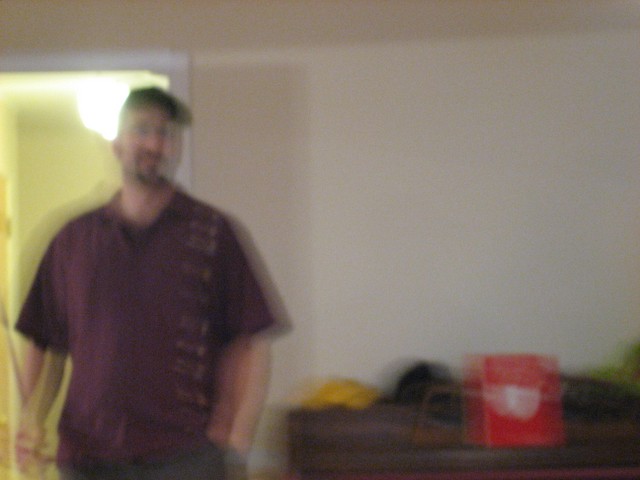In this rectangular, portrait-oriented photograph, a Caucasian man stands on the left side, looking outward. He sports a goatee and a baseball cap and is dressed in a short-sleeve purple shirt paired with dark brown pants. His left hand is tucked into his pocket while his right hand rests at his side. To his right, a dresser sits against a white wall, adorned with various objects in red, white, yellow, and black hues. Behind the man, a doorway is illuminated by a light above, casting a warm yellow glow in the background. The image is slightly blurred, adding a sense of movement or unsteady focus to the scene.